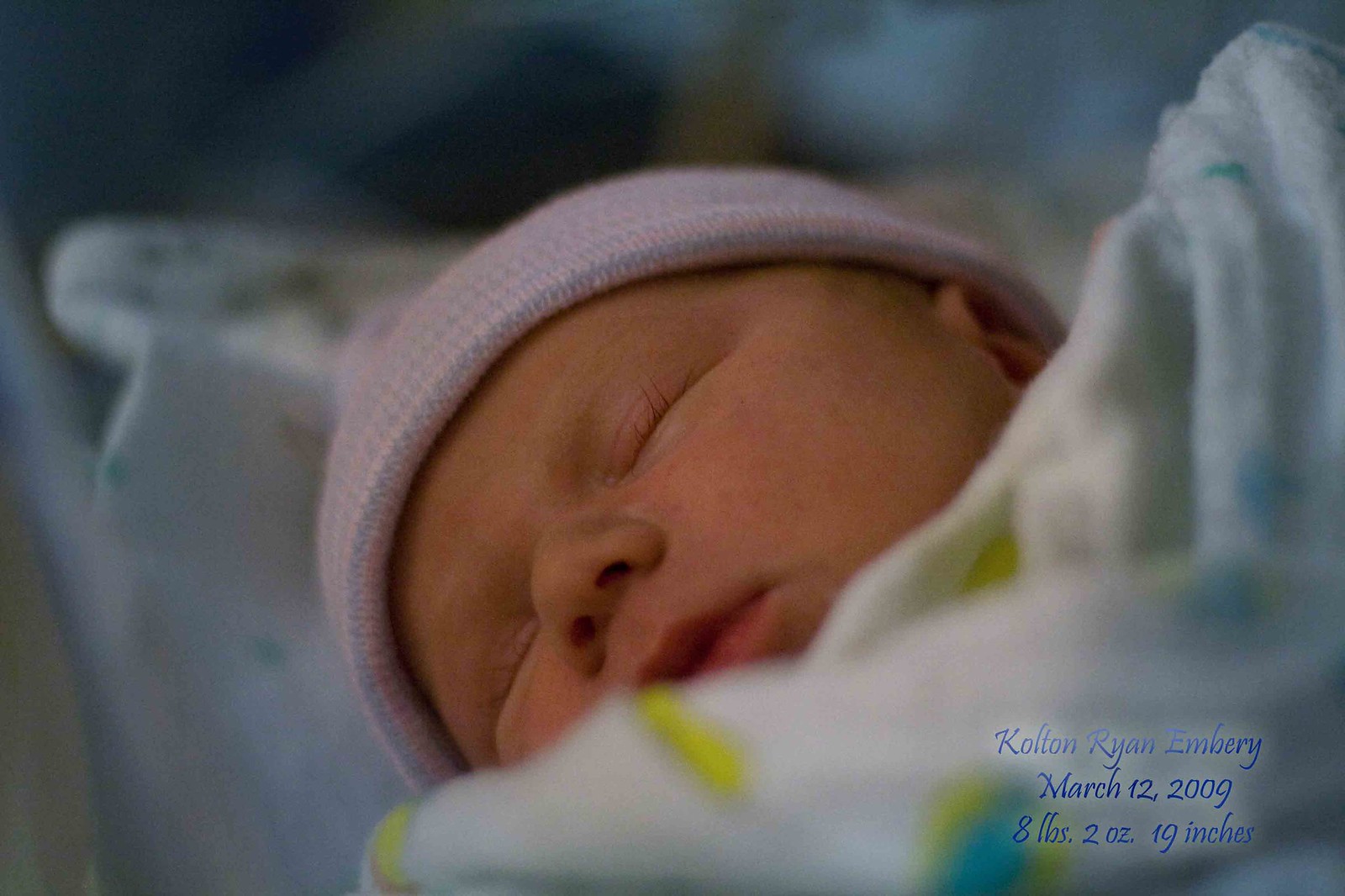This is an endearing close-up photograph of a serene, newborn baby sleeping peacefully. Positioned centrally in the image, the baby is lying on its right side, displaying a delicate face with closed eyes, a small nose, and slightly parted lips. The baby, presumably very young and quite tiny, is wearing a pinkish cap adorned with some white and blue accents. Its left ear is visible towards the middle top of the picture, and you can notice the baby’s long eyelashes adding to the cuteness. The baby is warmly wrapped in a mostly white blanket with hints of green and blue, enveloping the body and leaving only the face exposed. 

The background is softly blurred, creating a soothing and focused frame around the infant’s features. Along the left side, part of a white blanket that the baby is lying on can be seen. At the bottom right-hand corner of the image, there is blue writing that reads: "Colton Ryan Embry," followed by the details "March 12, 2009, 8 pounds, 2 ounces, 19 inches." The overall impression is one of tranquility and newness, capturing an adorable and tender moment of the freshly born baby.